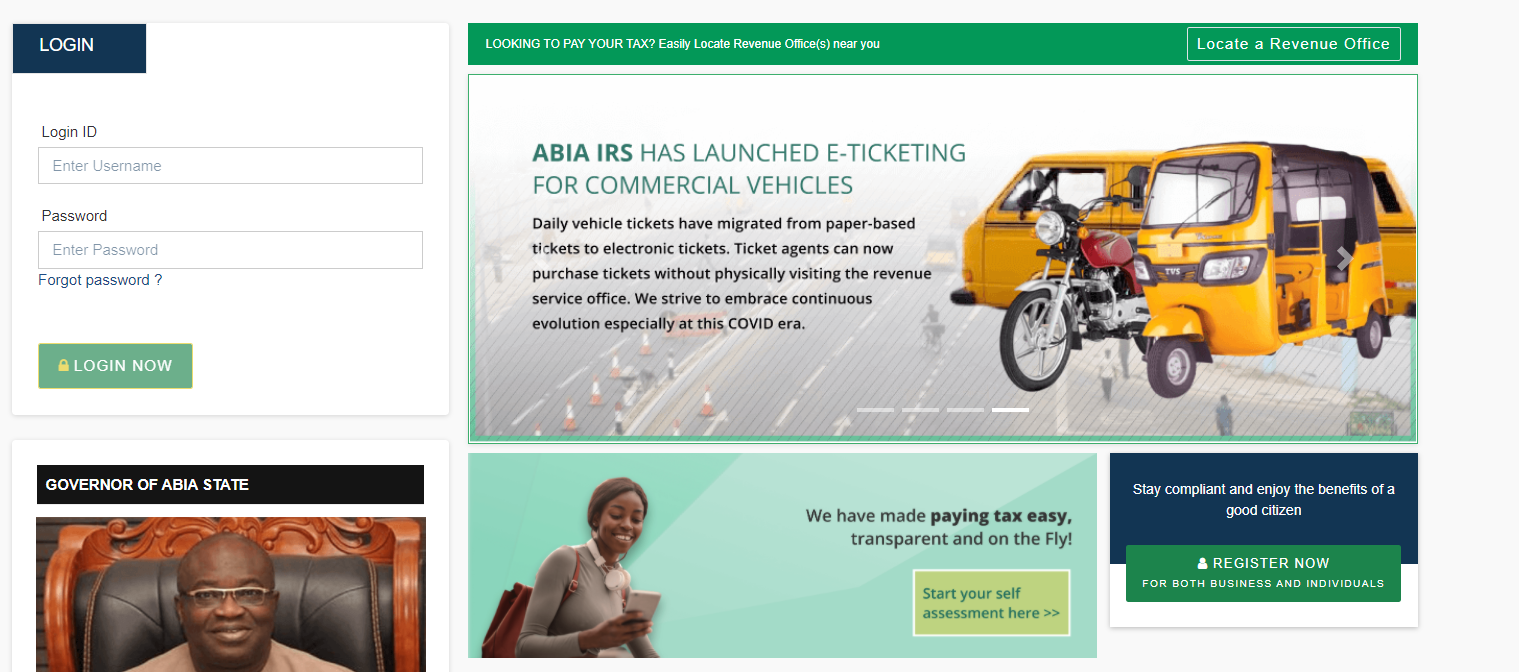**Detailed Descriptive Caption:**

The image features the login page for the ABIA IRS (Internal Revenue Service) portal. On the left side of the page, there is a vertical panel that serves as a navigation menu. Centrally positioned are the login fields: the first entry field, labeled "Enter Username," is followed by another field for the password input labeled "Enter Password." Below these fields is a blue button marked "Login." Adjacent to these, there's a "Forgot Password?" link for user assistance.

Directly beneath the login area, a green button to log in stands out within the interface. Further down is a portrait of an African gentleman, identified as the Governor of ABIA State. He is seated on an intricately carved wooden chair adorned with a plush leather seat. The Governor is bald, wearing sophisticated glasses and a beige jacket.

On the right side of this portrait, a green header poses the question, "Looking to pay your tax early?" Below this header, there's a section discussing revenue services, accompanied by a button labeled "Locate Revenue Office." 

A photograph depicting a van, motorcycle, and a tuk-tuk is displayed, highlighting the message: "ABIA IRS has launched ticketing for commercial vehicles. Daily vehicle tickets have migrated from paper-based to electronic tickets, enabling ticket agents to purchase them without visiting the revenue service office physically. We strive to embrace continuous evolution, especially in this COVID era."

Beneath this photograph, there is a smaller panel featuring a woman looking at her phone, with text announcing, "We've made paying tax easy, transparent, and on the fly." 

Towards the bottom right of the page, a blue section urges, "Stay compliant and enjoy good benefits as a good citizen," paired with a green button that says "Register Now."